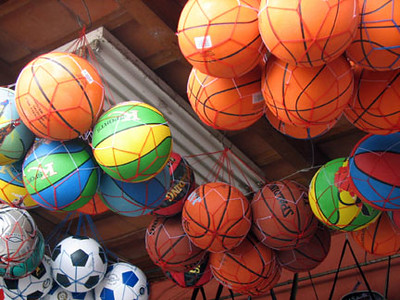The image depicts a colorful and somewhat low-resolution photograph taken from below, looking up at a ceiling covered in wooden rafters that are partly visible. Sunlight illuminates the scene, which features a variety of basketballs and soccer balls hanging from the ceiling in netting. The basketballs are stored in red and white nets, with some nets holding traditional orange and dark brown basketballs, while others contain more vibrant basketballs with stripes of red, blue, green, and yellow. One basketball notably resembles a Superman design. The soccer balls, found at the bottom left corner of the image, are held in blue nets and come in classic black-and-white designs as well as blue-and-white variants. A rectangular, gray fluorescent light fixture extends from the top left towards the center of the image, contributing to the utilitarian feel of the space, which seems reminiscent of a sporting goods store or a sports equipment storage area.